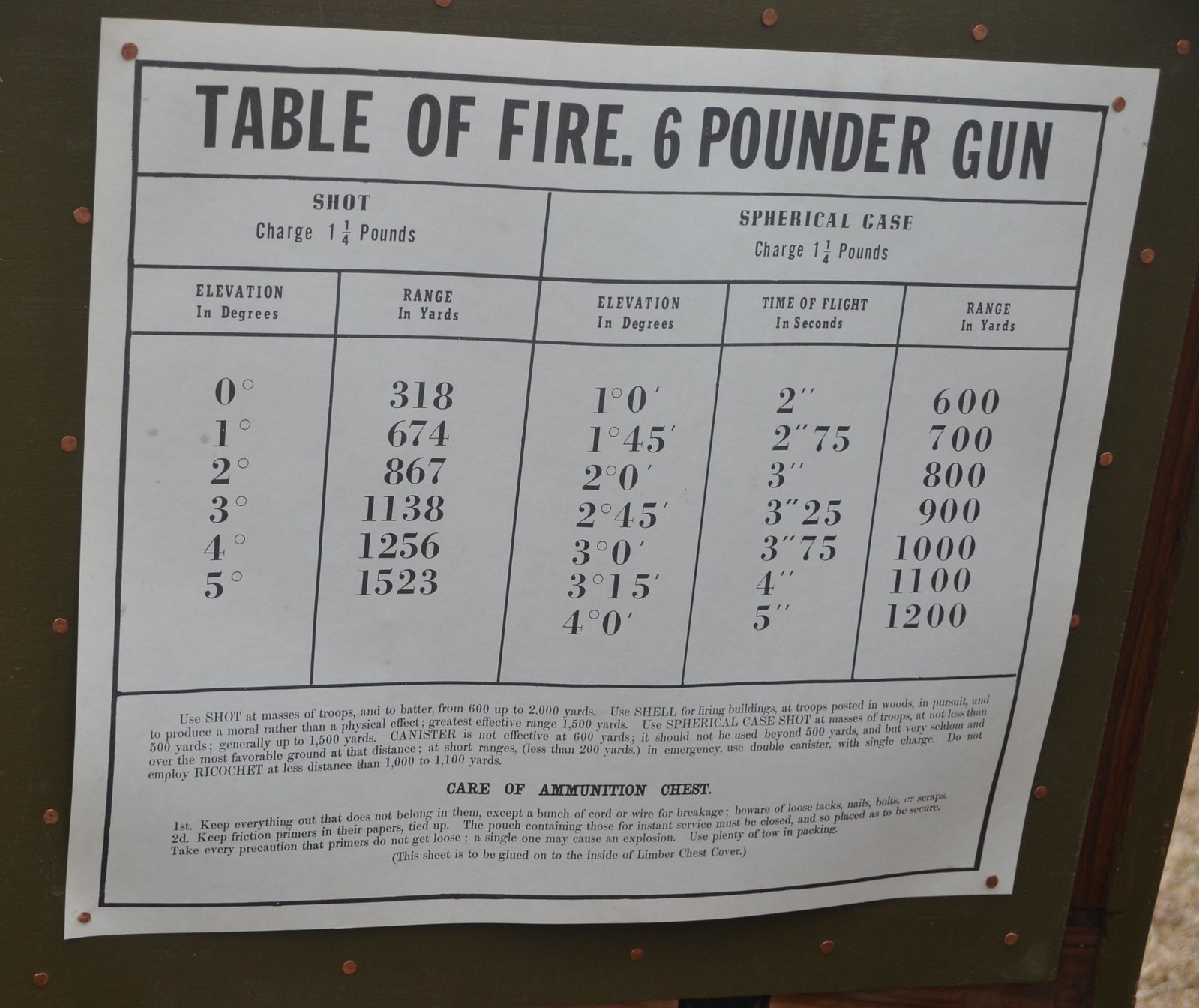The image features a piece of paper pinned to a wooden notice board, displaying a detailed table of fire for a six-pounder gun. The paper has a clean white background with black text and a thick black border surrounding the content. At the top, the heading reads, "Table of Fire, Six Pounder Gun." The table is divided into two primary sections, each with its own subheadings and columns.

On the left side, the section labeled "Shot" includes the subheading "Charge, £1.25." This section contains two vertical columns: "Elevation in Degrees" on the left and "Range in Yards" on the right. The data within this section lists various elevations (from 0 to 5 degrees) paired with their corresponding ranges (318 to 1523 yards).

On the right side, under the heading "Spherical Case" and also "Charge, £1.25," there are three columns: "Elevation in Degrees," "Time of Flight in Seconds," and "Range in Yards." This section details various elevations and their associated times of flight and ranges, such as "1 degree 0, 2 seconds, 600 yards" and ranges up to "4 degrees 0, 5 seconds, 1200 yards."

Below the table are two paragraphs of text pertaining to the care of ammunition, emphasizing the maintenance of the ammunition chest. The paper is affixed to the board with pins.